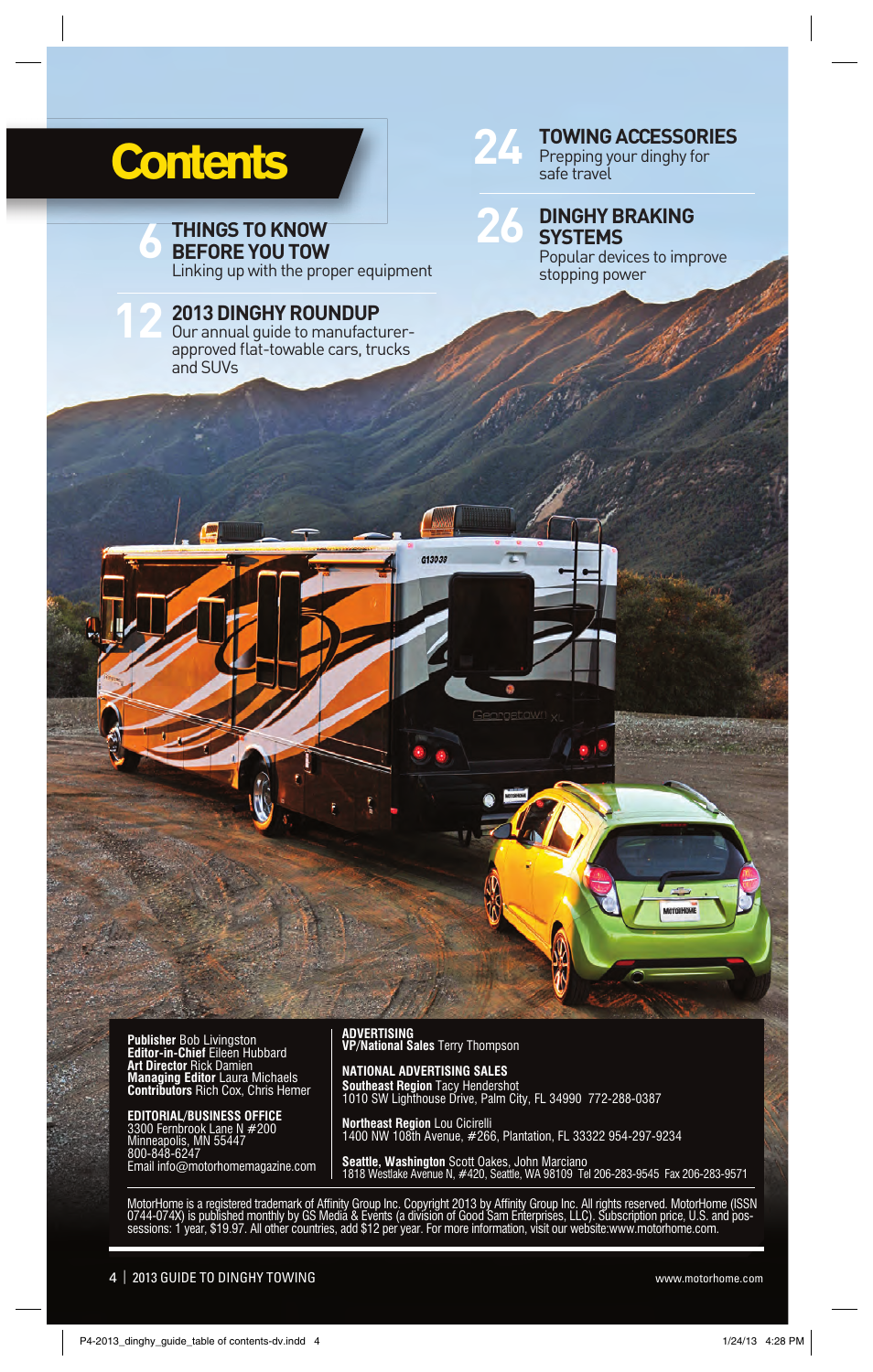The image is a screenshot, possibly from a cell phone, showcasing a camping scene that appears to be a page from an online magazine. At the center, an RV, painted with swirls of orange, white, brown, and black, travels to the right. The RV is set against a backdrop of brown mountains partially covered in green vegetation, and is situated on an open dirt field devoid of any grass.

Towed behind the RV is a small, fluorescent green Chevrolet, resembling a bug in its shape. The Chevrolet is connected to the RV, suggesting that it is being towed.

The text overlaying the image is an informative guide about towing. The headings and page numbers provided are:

- "Contents: Six Things to Know Before You Tow, Linking Up with the Proper Equipment" (Page 12)
- "213 Dinghy Roundup, Our Annual Guide to Manufacturer Approved Flat Towable Cars, Trucks, and SUVs" (Page 24)
- "Towing Accessories, Prepping Your Dinghy for Safe Travel" (Page 26)
- "Dinghy Braking Systems, Popular Devices to Improve Stopping Power" (Page 26)

This suggests the image is part of a magazine issue focusing on towing dinghies. 

A black box within the image contains information too tiny to read, but at the very bottom, one can make out, "213 Guide to Dinghy Towing" and the website "www.motorhome.com," reinforcing that this is a guide on towing.

Additional text at the bottom reads, "p4-2013-dinghy-guide-table of contents.dv.indd.4". To the bottom right, there's a timestamp: "1/24/13 at 4:28 PM". No additional information is present.